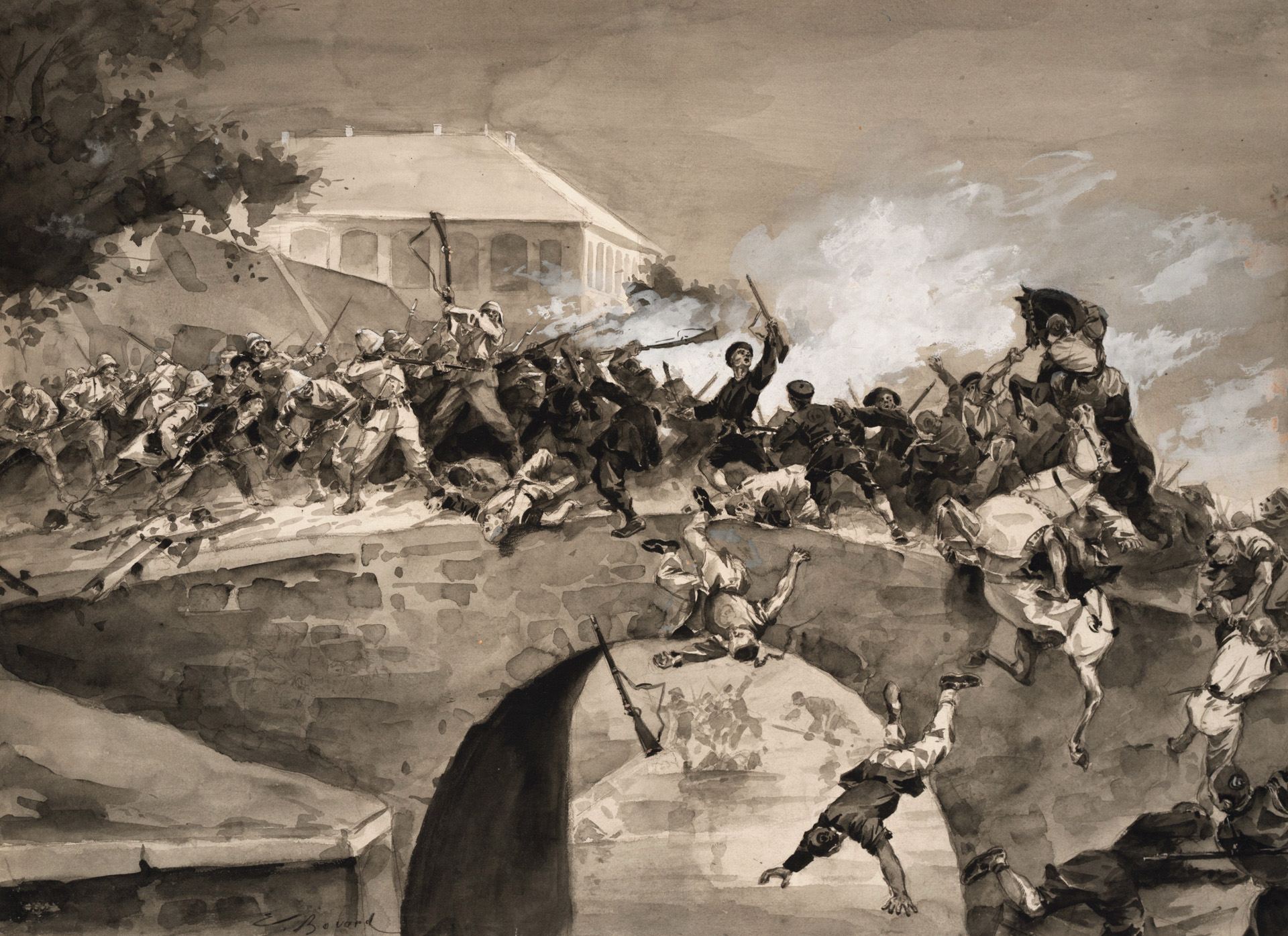This black and white image, likely a painting or drawing reminiscent of a lithograph without traditional lines, dramatically depicts a chaotic and fierce battle on an arched stone bridge without any rails. The bridge, densely packed with around 40 to 50 clashing combatants, showcases soldiers wielding swords and long arms, with some brandishing guns. Amidst the turmoil, several figures are depicted falling or clinging to the edges of the bridge, including a horse tumbling off the side. The bridge stretches over a waterway or trench, and in the upper left corner of the piece, there's a large white building with arched windows and a peaked roof, partially obscured by a nearby tree. The monochrome palette and historical elements suggest a scene from an older era, potentially even reminiscent of a battle from the Revolutionary War. The sky, filled with puffs of white, adds to the enigmatic atmosphere, leaving viewers to ponder whether these are clouds or smoke from the conflict below.